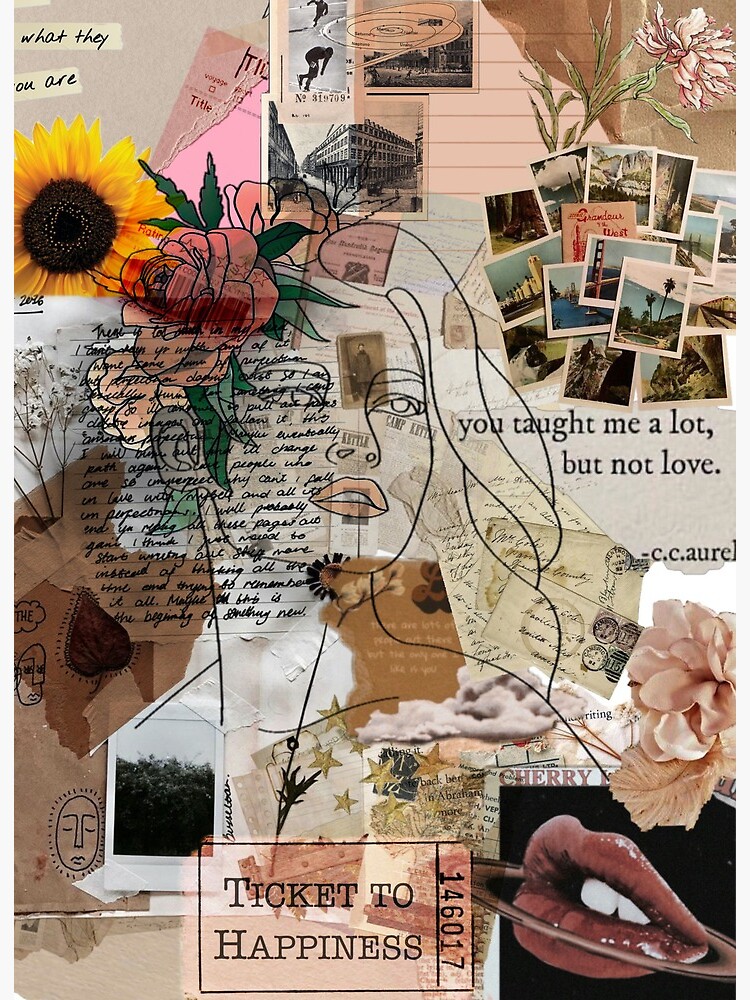This intricate collage style artwork features a central drawing of a woman with light pink lipstick, facing to the right with her lips slightly parted. Overlaid and interwoven with this central figure are numerous abstract and concrete elements, creating a rich and evocative visual tapestry. Prominent among these elements are various flowers, including a vivid yellow sunflower with a black center and a pink rose doubling as a hair ornament. 

The collage is peppered with vintage-looking stamps and postcards, contributing to its nostalgic feel. Quotes and phrases are scattered throughout, the most notable being "You Taught Me A Lot But Not Love" attributed to C.C. Aurel, and a pink ticket stub labeled "Ticket to Happiness" with the number 146017. There are disembodied red lips drawn in a pop-art style at the bottom right, along with other smaller photographs and images. The background and many items lean towards a color palette of pinks, beiges, and yellows, adding warmth and cohesiveness to the piece.

In essence, this artwork is a carefully constructed collage that serves as both a vision board and a deeply personal narrative, interlacing inspirational images, quotes, and drawings to resonate emotionally with its viewer.